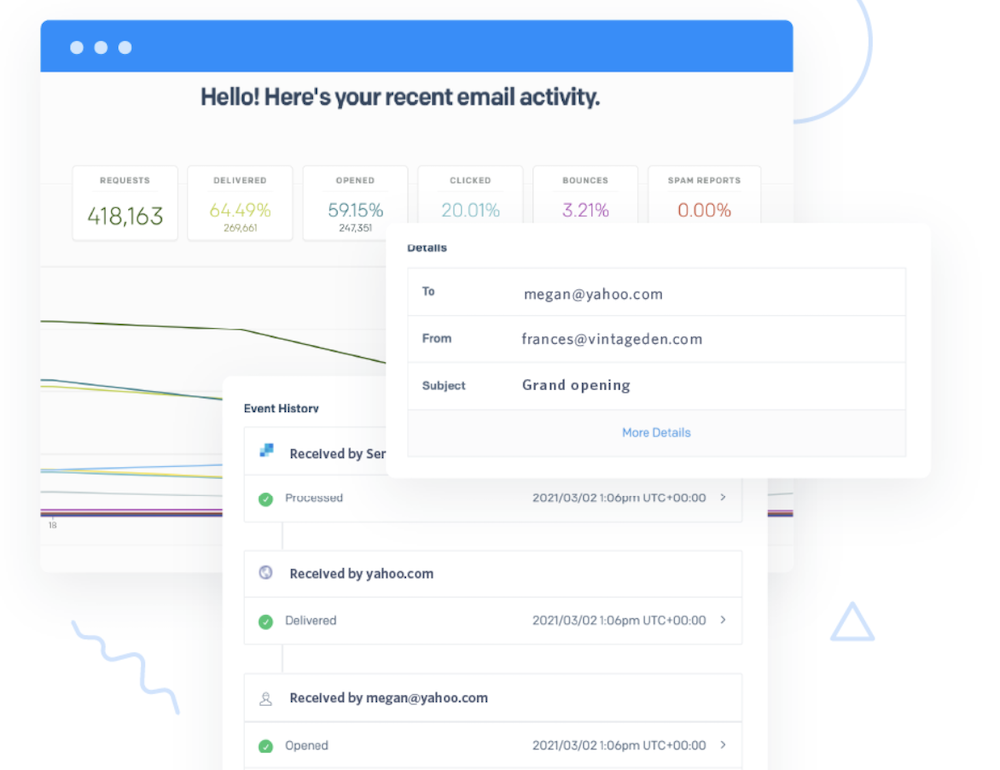This is a detailed caption:

---

The screenshot captures an email analytics dashboard with a prominent blue rectangle banner at the top of the page, set against a white background. Below the banner, three overlapping windows are open, displaying various data metrics and information. 

In the first window, the email activity summary reads:
- Request: 418,163
- Delivered: 64.49%
- Opened: 59.15%
- Clicked: 20.01%
- Bounces: 3.21%
- Spam Reports: 0

A partially obscured bar graph visually represents each of these percentages.

The second window provides specific email details:
- Recipient: Megan at Yahoo
- Sender: FrancisVintageDen.com
- Subject: Grand Opening
- Additional information link: "More details" in blue text
- Received details: Delivered on 03-02-2021 at 1:06 PM

The third window confirms the email reception and interaction:
- Received by Megan with a green checkmark indicating the email was opened
- Opened timestamp: 03-02-2021 at 1:06 PM, suggesting immediate engagement upon delivery.